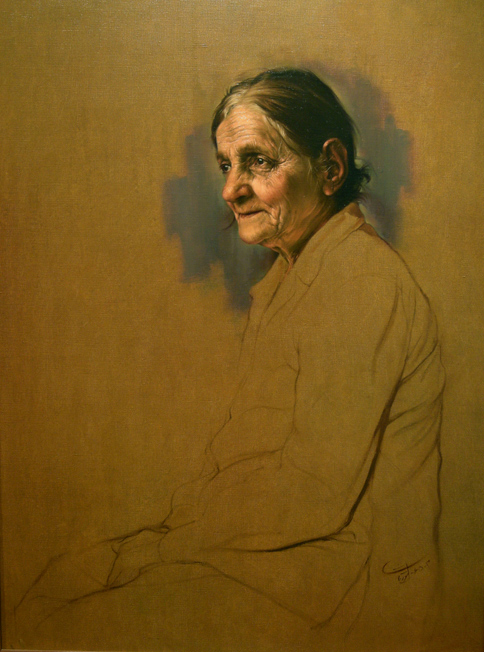This is a vertically aligned rectangular painting of an older woman, likely in her late 70s or early 80s. Her hair, predominantly gray with white streaks, is pulled back into a ponytail or bun. The side profile shows her looking to the left with a serene expression, her mouth slightly open—not quite smiling yet not frowning. Her dark eyes convey a sense of longing, and her face is marked with wrinkles and subtle blush on the cheeks, adding a touch of color to her otherwise pale complexion.

The backdrop is a solid medium brown, with textural elements like gray splotches and black smudges providing depth behind her head. She’s dressed in a collared top and pants that seamlessly blend with the monochromatic brown palette of the background. Her hands are folded on her lap, and the view extends to her knees, from which the image trails off into the lower right-hand corner. The lower back of the painting bears a cursive artist’s signature, though it remains indecipherable. The overall composition is rendered on a yellowish-brown canvas, with the detailed depiction of her face contrasting against the more sketch-like representation of her body below the neck.